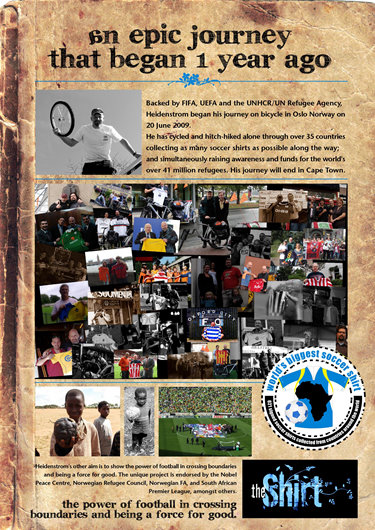The image appears to be a page from a brochure or a book with a worn, light and dark brown cracked background. At the top, in black text, it says, "An epic journey that began one year ago," with the 'A' in "Ann" printed backwards. Below, there's a blue squiggly line in the middle. On the left side, there is a black-and-white picture of a man wearing a white shirt and black hat, holding a bicycle tire with his left arm while his right arm rests against a wall. This image has a gray background.

Next to the photo, there is black text stating: "Backed by FIFA, UEFA, and the UNHCR/UN Refugee Agency, Heather Heidenstrom began his journey on bicycle in Oslo, Norway on 20 June 2009. He has cycled and hitchhiked alone through over 35 countries, collecting as many soccer shirts as possible along the way, while simultaneously raising awareness and funds for the world's over 41 million refugees. His journey will end in Cape Town."

Below this text, there's a large collage of square photos, densely packed, mostly featuring people. In the bottom right corner of the collage, there is a circle with a white background that says "World's Biggest Soccer Shirt." Underneath the circle, there is an image of a blue soccer shirt with a black depiction of the African continent and a soccer ball below it.

At the very bottom, there are three additional pictures: on the left, two young Black men; in the middle, a small Black boy in a black-and-white image; and on the right, a photo resembling a soccer stadium. Below these, some black text reads, "The power of football in crossing boundaries and being a force for good." In the bottom right corner, there is a blue square with white text that reads, "The Shirt."

The overall theme resembles a beaten-up notebook, emphasizing a journey and the unifying force of football.